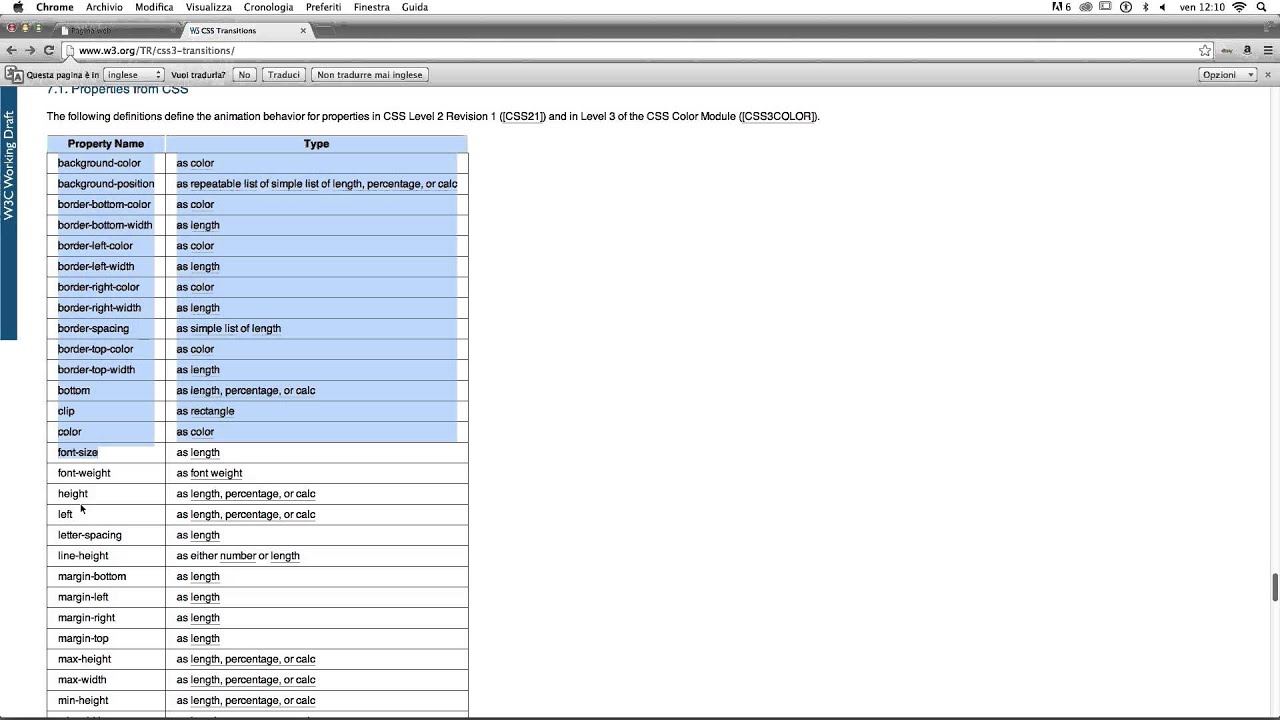A screenshot captures a computer monitor displaying the W3C (World Wide Web Consortium) documentation for CSS transitions. The URL in the search bar reads "www.w3.org/TR/css3-transitions," and a notification below offers translation options in Italian, with phrases like "questa pagina in inglese" and "vuoi tradurla" visible. The main content area features section "7.1 Properties from CSS," introducing definitions for animation behavior properties in various CSS levels, including CSS 2.1 and CSS3 Color Module.

The visible portion of the content includes a detailed chart outlining CSS property names and their respective types. The listed properties include:

- Background color: color
- Background position: repeatable list of lengths, percentages, or calculations
- Border properties (bottom, left, right, top) with their color and width attributes
- Letter spacing: simple list of lengths
- Bottom, clip, color, font size, font weight, height, left: various types including length, percentage, or calculation
- Line height: either number or length
- Margin properties (bottom, left, right, top): length
- Max height and width, min height and width: length, percentage, or calculation

A dark blue vertical border on the left side of the screen prominently features the "W3C" logo.